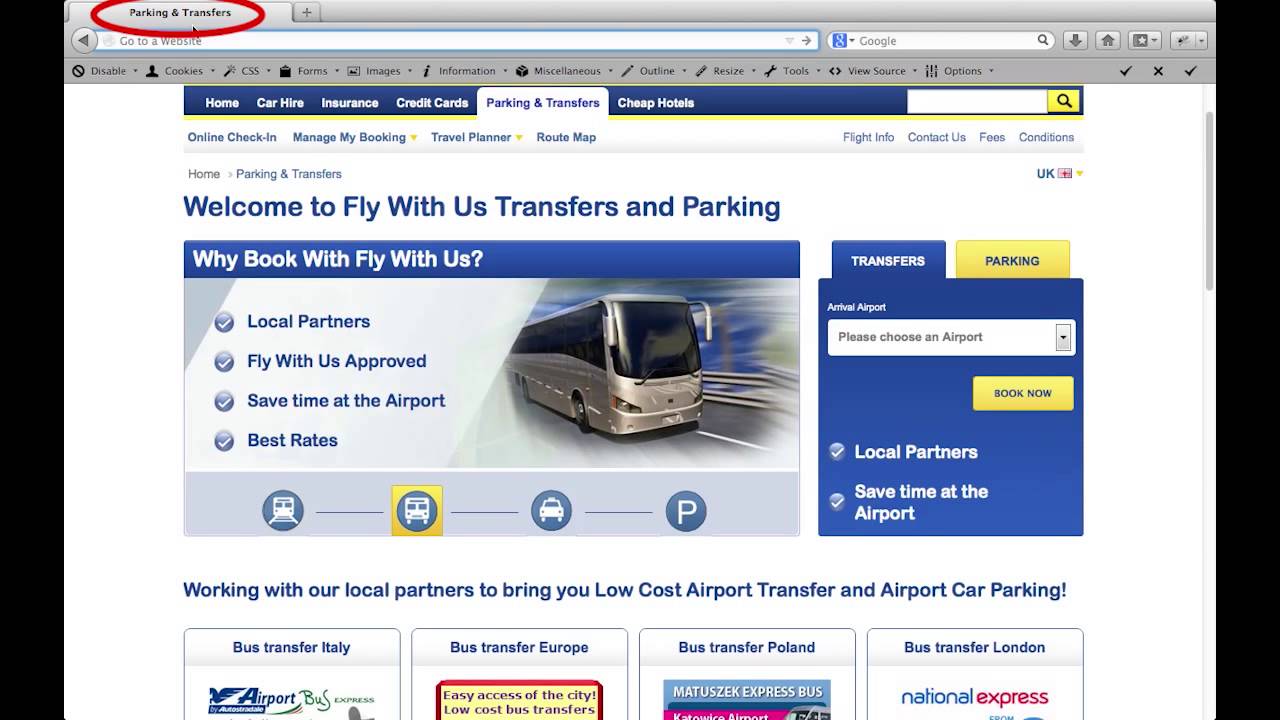The web page features a symmetrical design with solid black bars framing each side, and a clean white background. At the top, there is a light gray web browser interface, which includes several elements. 

In the upper left corner of the browser, an open tab labeled "Parking and Transfers" in black text is highlighted with a bright red oval outline and a black cursor prominently placed inside the oval. Below this, a web URL box, outlined in light blue, contains black text reading "Go to a Website." The box also features a dark gray play button on the left and light gray and dark gray arrows on the right. Alongside, a secondary search box, marked by a blue and white Google icon, displays light gray text that reads "Google" and a dark gray magnifying glass icon on the far right. Adjacent to these elements are four square-shaped icons: a dark gray downward arrow, a house icon with a pointed roof and light gray door, a gray box with a light gray star, and an indistinct symbol that resembles an insect. Each icon is accompanied by a light gray downward arrow.

The main body of the page is dominated by a white background accentuated with dark blue and yellow highlights. A bold header at the top announces, "Welcome to Fly With Us Transfers and Parking." Below, a blue-bordered section with white text poses the question, "Why Book With Fly With Us?" Accompanying this text are four circular light blue buttons, each marked with a white checkmark and labeled with dark blue text: "Local Partners," "Fly With Us Approved," "Save Time at the Airport," and "Best Rates." 

Adjacent to this section is a computer-generated image of a sleek, silver metallic bus. Beneath it, bright blue text declares, "Working With Our Local Partners to Bring You Low-Cost Airport Transfer and Airport Car Parking."

To the right of this image, a bright blue square box houses two tabs: a white text "Transfers" tab on a blue background, and a "Parking" tab in yellow with blue text. Inside the box, the prompt "White Arrival Airport" leads to a drop-down menu featuring the placeholder text "Please Choose an Airport." Below this menu is a yellow button with blue text stating "Book Now." On the lower left, two circular light blue buttons marked with white check marks are labeled "Local Partners" and "Save Time at the Airport."